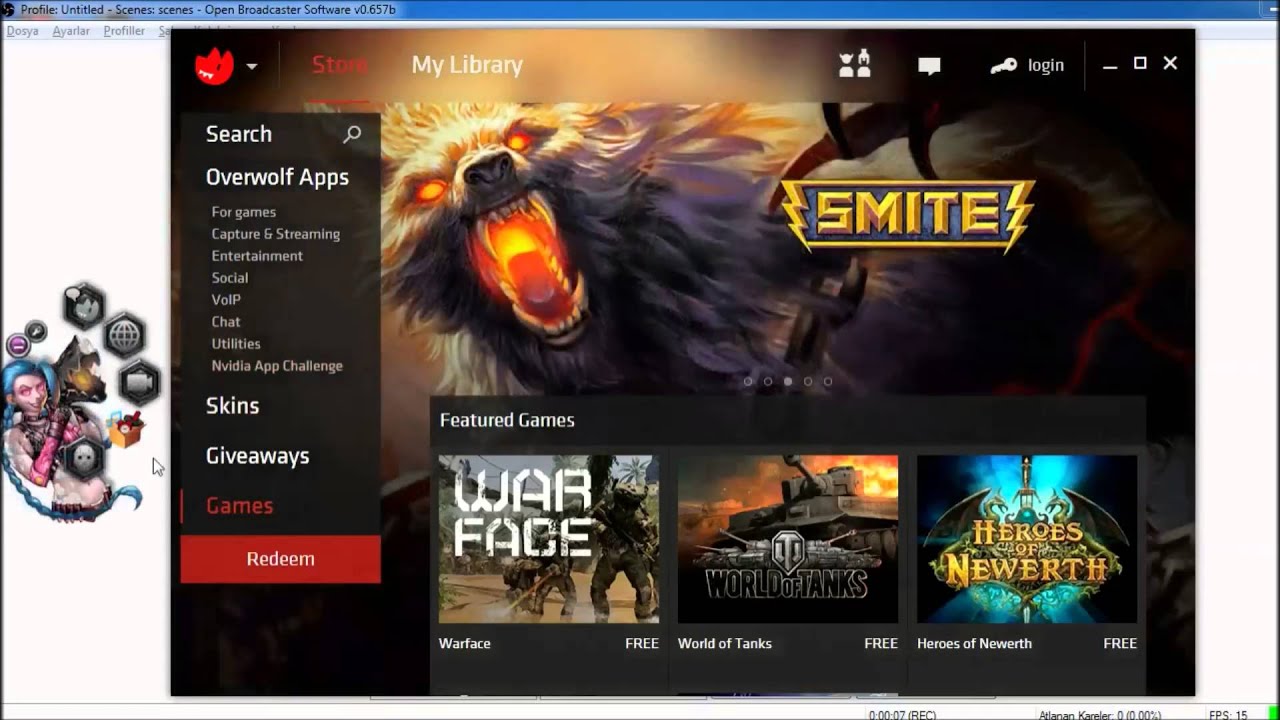This image showcases the interface of a customer's login profile within Open Broadcaster Software (OBS). At the top of the screen, the menu options are displayed from left to right, starting with 'Store' and followed by 'My Library'. There are four distinct icons present: a chat button, a key image, a login button, and a search option on the left side along with a rectangular search box.

Listed from top to bottom on the left side are categories for various app types: 'All', 'Apps', 'Games', 'Capture and Streaming', 'Entertainment', 'Social', 'VOIP', 'Chat', 'Utilities', and the 'NVIDIA App Challenge'. This section concludes with options labeled in bold for 'Skins', 'Giveaways', and 'Games', along with a 'Redeem' option at the bottom.

On the far left side of the screen, outside the OBS gaming software portal, are clickable game icons featuring specific games. One prominent game displayed is 'SMITE', characterized by a logo that includes an image of a wolf with fiery eyes set against its backdrop.

At the bottom of the screen, there's a rectangular section dedicated to 'Featured Games'. The games listed here from left to right include 'Warface', 'World of Tanks', and 'Heroes of Newerth', all of which are currently priced as free.